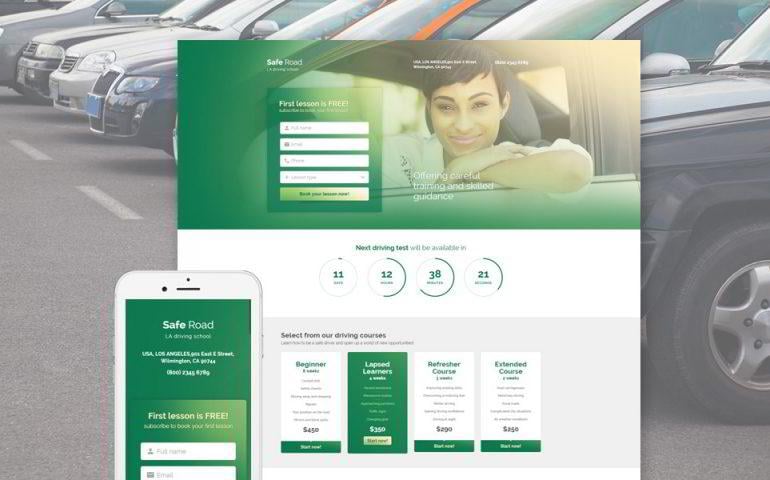This image captures a tightly zoomed-in view of a parking lot, focusing on a row of cars all facing towards the left, neatly lined up. White parking lines are visible in front of the vehicles, segmenting the lot. Dominating the majority of the image is a semi-transparent overlay with "Safe Road" displayed at the top.

Superimposed on the parking lot scene is a green-tinted picture of a woman sitting in a car, looking out the driver's side window at the camera. Her elbow rests nonchalantly on the window ledge. Above and below her image, there is some text, though it's not clearly readable. To her left, there’s a blurry box with text that is indecipherable, which contains four input fields.

Below this image, four circles are arranged horizontally, each containing text. From left to right, the circles display the numbers 11, 12, 38, and 21. At the very bottom of the image, four boxes filled with text are visible, adding further information to this composite visual message. The overall tone and layout suggest a focus on safe driving or road safety awareness.